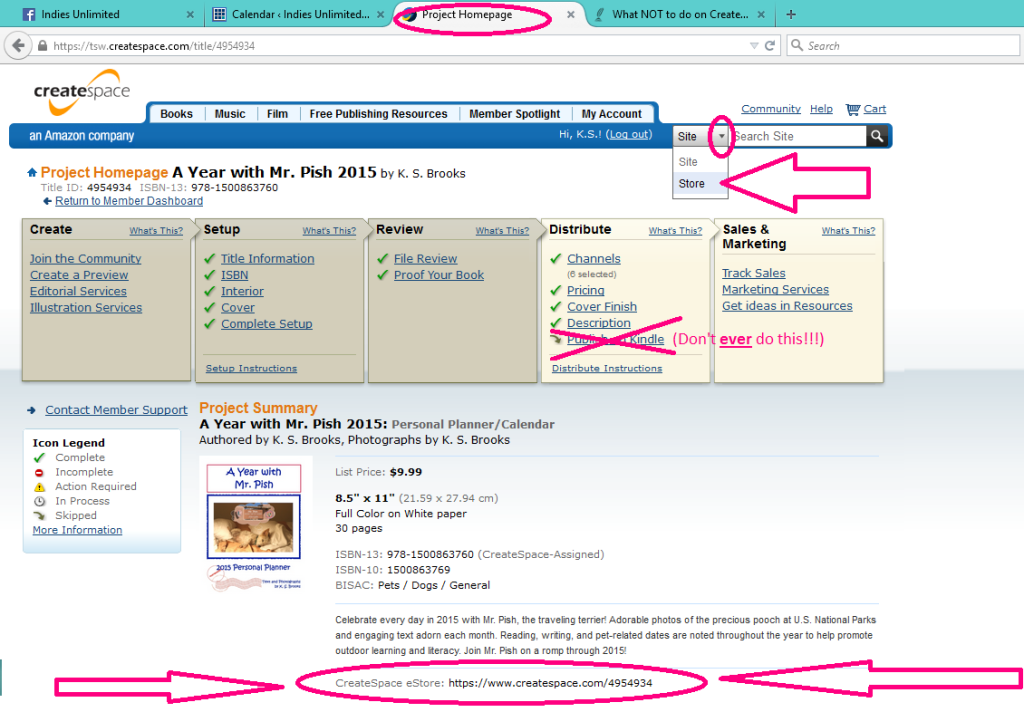The screenshot captures a web page within a browser window. The top border of the browser is adorned with a turquoise hue, and the active tab, labeled "Project Homepage," is highlighted with a pink oval. Just below the tab, the URL bar displays "tsw.createspace.com/title/4954934."

The main content of the web page begins with the CreateSpace logo located at the upper left corner. The logo features "create" in bold lowercase letters and "space" in light gray, with both words amalgamated. Adjacent to this text, a gold squiggly line forms part of the company logo. Below the logo, a blue menu bar provides navigation options. To the left, it states "an Amazon company" in white. The menu items themselves—"Books," "Music," "Film," "Free Publishing Resources," "Member Spotlight," and "My Account"—are presented in black font against a very light blue background.

Directly beneath the menu, "Project Homepage" is written in a gold font. Below this, a heading in black font reads "A Year with Mr. Pish 2015," authored by K.S. Brooks in smaller gray text. The page features five function buttons—"Create," "Set Up," "Review," "Distribute," and "Sales and Marketing"—displayed as three gray boxes followed by two white ones. These buttons facilitate various self-publishing tasks through CreateSpace.

Further down, an image of the book project, "A Year with Mr. Pish 2015," is displayed, along with its list price of $9.99. The book's description reads, "Celebrate Every Day in 2015 with Mr. Pish," followed by additional details. At the bottom of the screenshot, the CreateSpace URL is circled in pink, with two arrows pointing towards it from opposite sides.